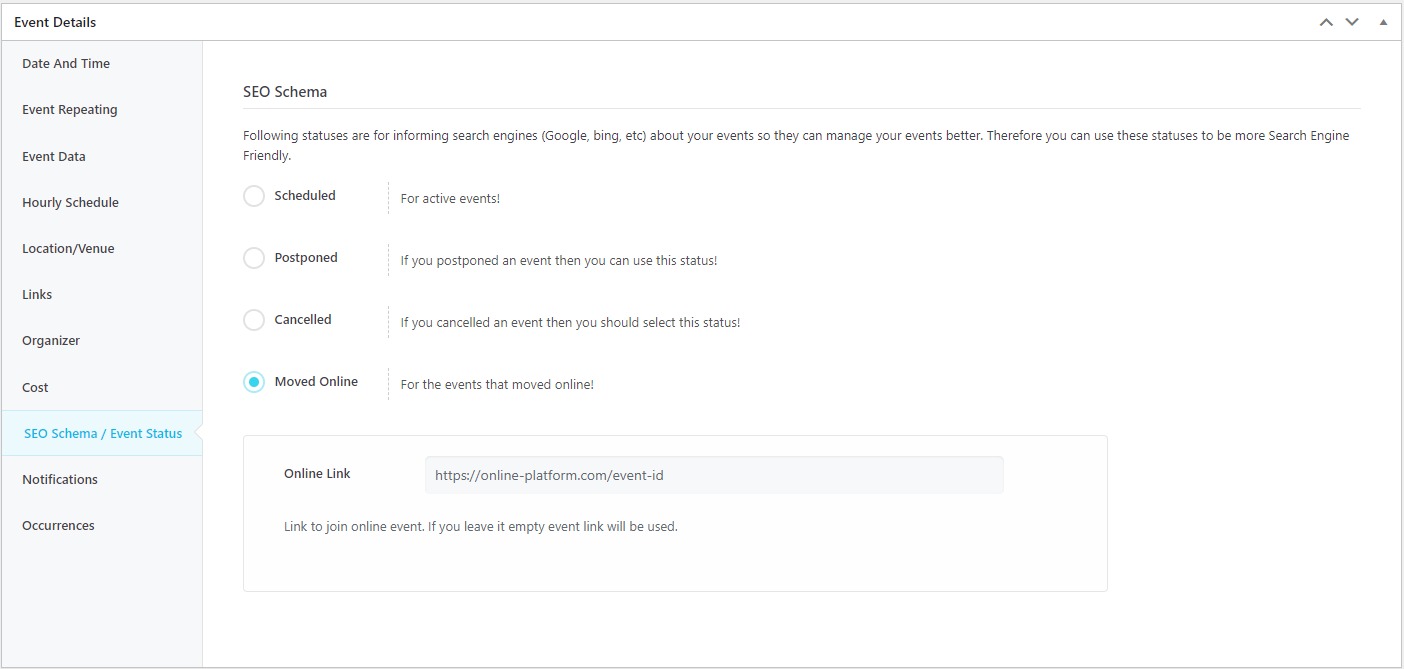This image depicts a detailed overview of event information on a white background with light black lettering. 

In the top-left corner, the title "Event Details" is prominently displayed. To the right, up and down arrows signify scrollable content. The subsequent items listed start with "Date and Time," followed by "Event Data," "Hourly Schedule," "Location/Venue," "Links," "Organizer," "Costs," and then "SEO Schema/Event Status" which is highlighted in blue. Below this, in black, it reads "Notification Occurrences."

On the right side, there is a detailed explanation about "SEO Schema" presented next to a gray line. This line includes the following note: "Following statuses are for informing search engines (Google, Bing, etc.) about your events so they can manage your events better. Therefore, you can use these statuses to be more search engine friendly."

Underneath, there are several circular status indicators. Each status is explained as follows:
- A circle indicating "Scheduled" for active events.
- "Postponed" indicates a rescheduled event.
- "Canceled" is used for events that have been called off.
- "Moved Online" is marked by a blue dot in its circle, indicating that the event has been switched to an online format.

Below this section, a light gray box contains the text "Online Link," and another gray box provides a URL: "https://online-platform.com/event-id." At the bottom, there is a note stating "Link to join online event. If you leave it empty, event link will be used."

Overall, the image provides a thorough breakdown of event details and how to optimize them for better search engine visibility.